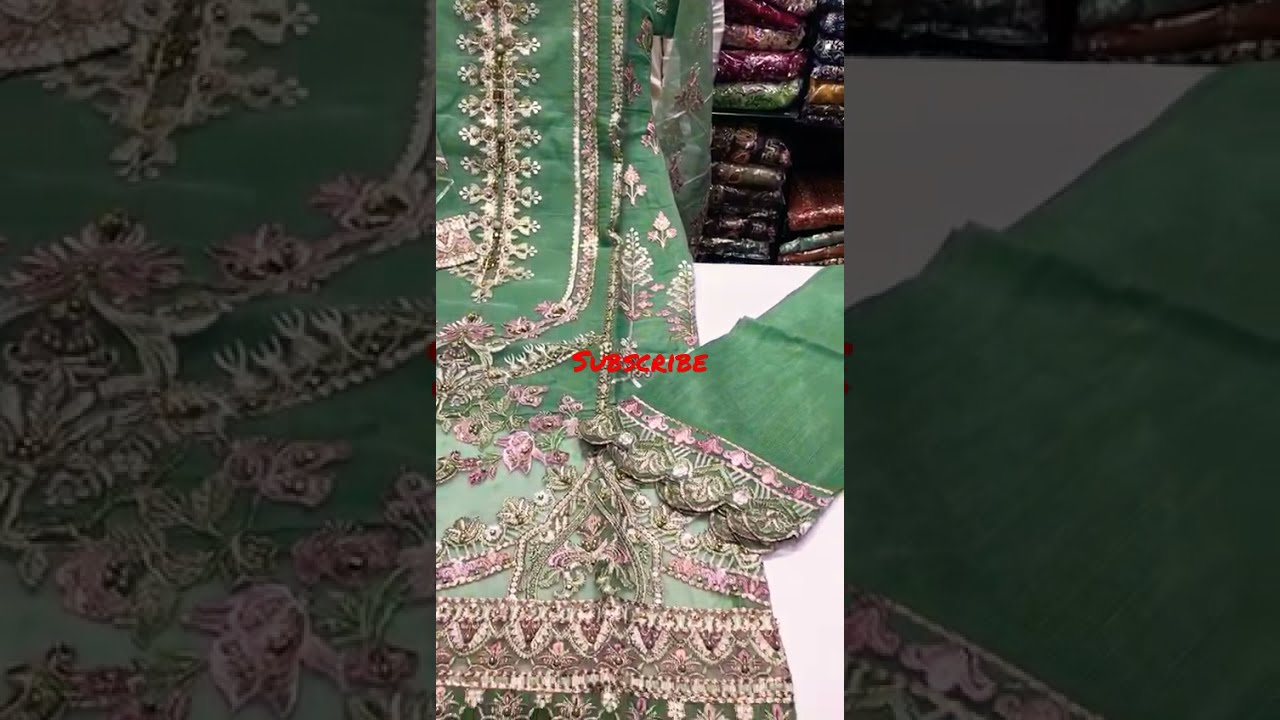The image consists of three equally sized panels, each depicting various views of an elaborate green fabric, likely part of an ornate dress or sari. The left panel shows a darkened close-up of this fabric, which features intricate purplish designs and elaborate stitching. The middle panel, which is more brightly lit, showcases the green material draped and laying on a white table. This fabric is richly decorated with delicate floral and gemstone embellishments, incorporating light rosy pink florals and clear crystal-like gemstones, along with lighter green leaves. The middle panel contains the word "SUBSCRIBE" in handwritten-style capital letters and reveals a background with numerous neatly stacked and folded fabrics in a closet-like area. The right panel mirrors the left with another darkened image of the green fabric, showing it at an angle from the upper right to the lower left. This panel also emphasizes the fabric's ornate end, replete with elaborate stitching.